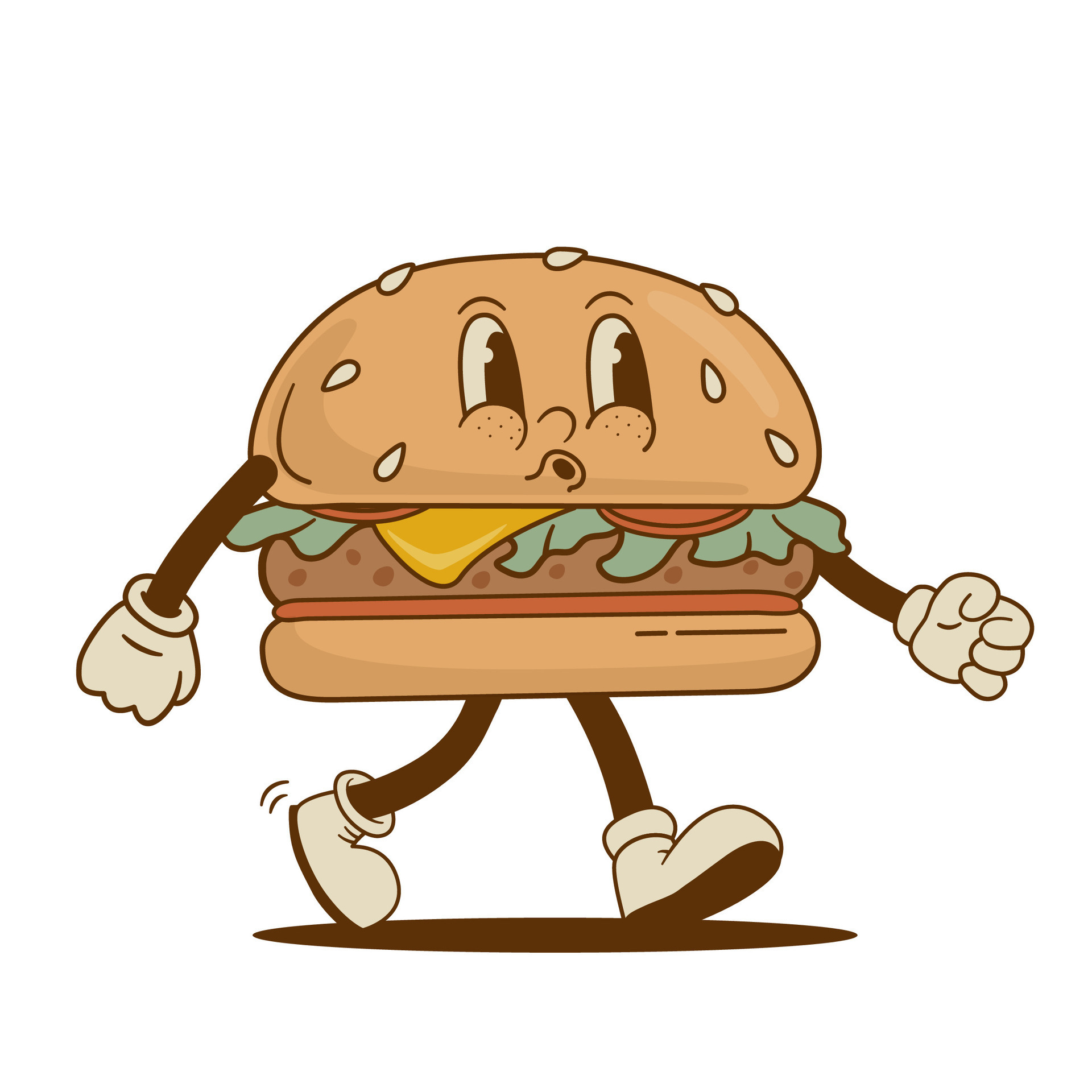This is an animated, cartoonish drawing of a cheerful, anthropomorphic hamburger walking to the right. Positioned centrally against a white background, the hamburger features a top bun dotted with white sesame seeds, and serves as the character's head, adorned with archway-shaped eyes, a small protrusion for a nose, and cheeks with black dots. The hamburger is whistling, suggested by the shape of its mouth. It has brown, thin arms with white gloves and brown, thin legs with white shoes. The left arm is extended downward and to the left, while the right arm extends downward and to the right. The left leg is firmly on the ground with the heel down and the foot partially lifted, while the right leg is raised slightly, positioned on its tiptoe. The body of the hamburger consists of a burger patty, leafy green lettuce, a slice of tomato, and yellow cheese, all situated between the top and bottom brown buns. A thin reddish band is visible under the patty, possibly part of the bottom bun. A brown disc beneath the feet likely represents the character's shadow, adding to the lively, dynamic feel of the scene.